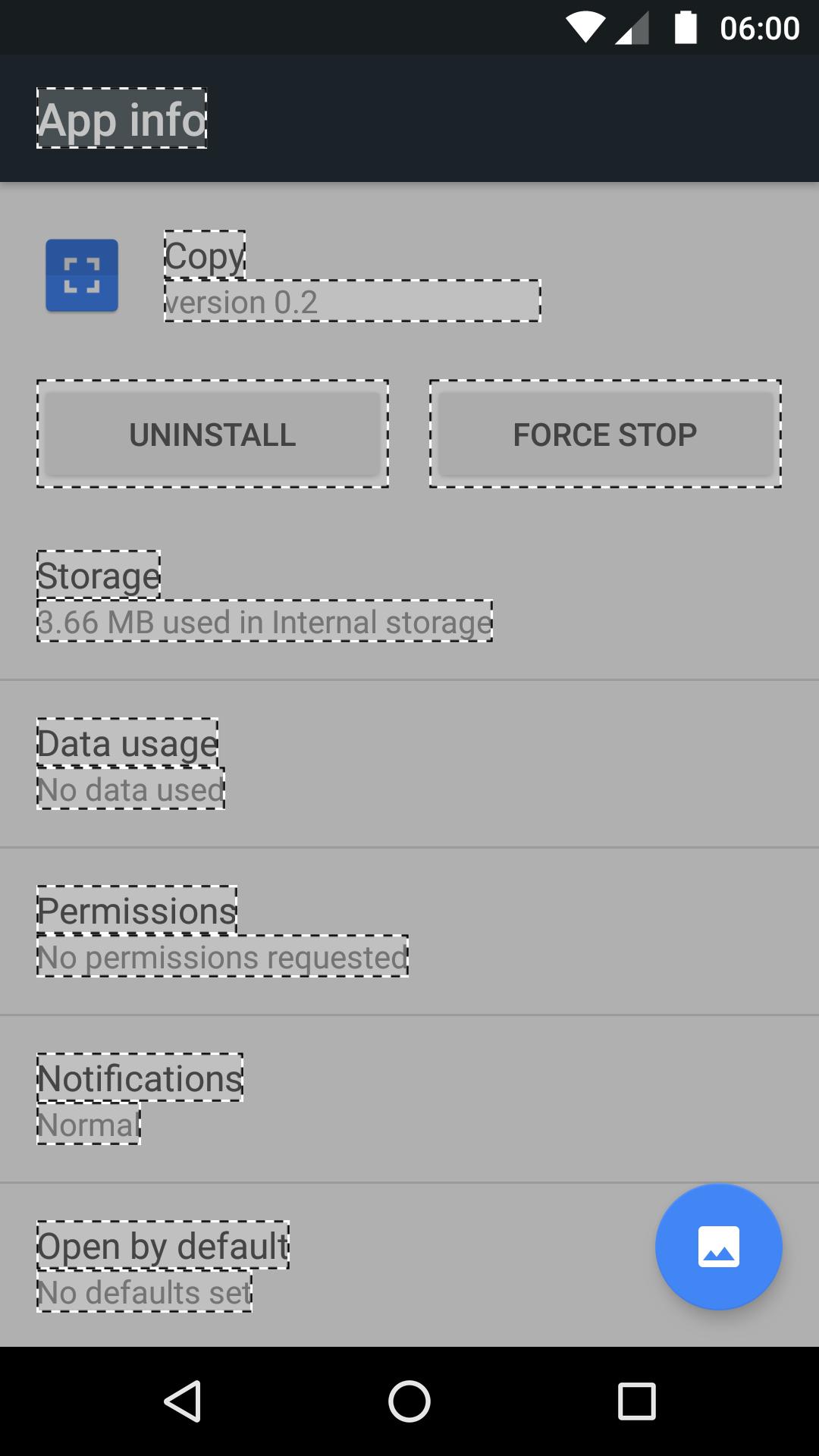This image displays the app information screen on a smartphone. At the top of the screen, the status bar shows a battery icon, signaling it is 6 o'clock. Below this, the heading "App Info" is highlighted in white text against a gray background, encased by a dashed line.

Directly beneath the header is the app's icon, a blue square featuring a smaller, open-frame silver square within it. Next to the icon, the text reads "Copy Version 0.2". Below this, there are two action buttons labeled "Uninstall" and "Force Stop".

Scrolling further down, the storage usage for the app is indicated as "3.66 MB used in internal storage". The data usage section reports "No data used". In the permissions area, it states "No permissions requested". The notifications section is marked as "Normal". The "Open by default" section mentions "No defaults selected" with the annotation "SEL".

At the bottom of the screen, there is a prominent blue button, and further down are three navigational icons that can be clicked for additional options.